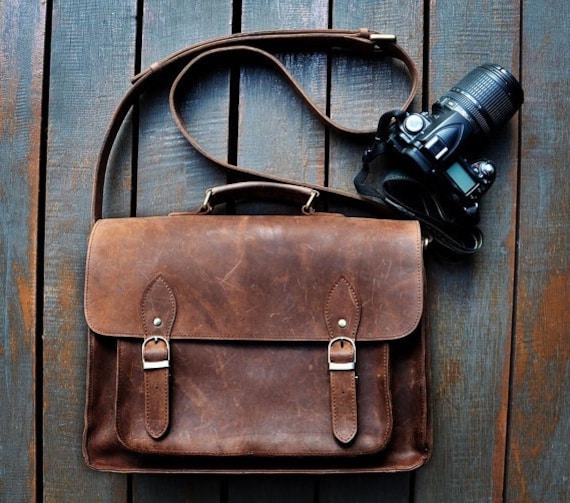The image captures a brown leather satchel and a sophisticated DSLR camera with a long lens, both set atop a weathered, slatted wooden surface partially painted blue. The satchel, exhibiting signs of wear and distress, features two buckle straps and both a handle and a longer strap for versatile carrying options. Nearby sits the camera, likely from the late 2000s to early 2010s, appearing well-maintained and possibly black and silver in make. The setting suggests an outdoor location such as a park bench, picnic table, pier, or boardwalk, evoking a rustic and worn ambiance that hints at frequent use and exposure to the elements, potentially in regions like Seattle or Jersey.